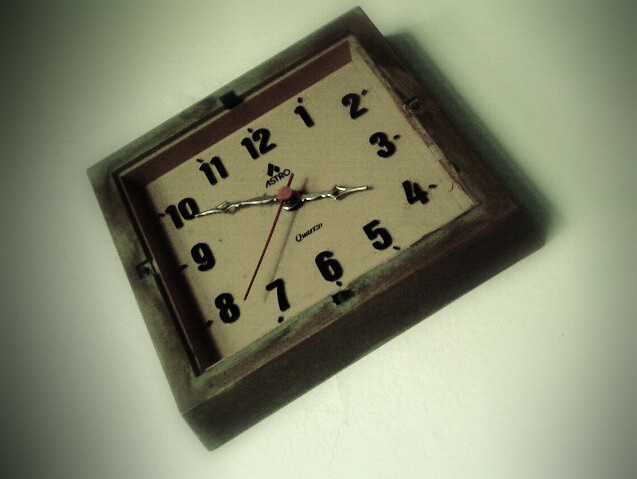Against a light gray wall that subtly transitions to a darker shade around the corners, a rustic, dark brown wooden clock is mounted, slightly askew. The clock's wood has a matte finish, emphasizing its vintage charm. Its face is a light brown color, with standard dark brown numerals marking the hours. The time is indicated by sleek silver minute and hour hands, while the second hand stands out in vivid red. The shadow of the clock is distinctly visible, particularly casting a pronounced silhouette on the right side.